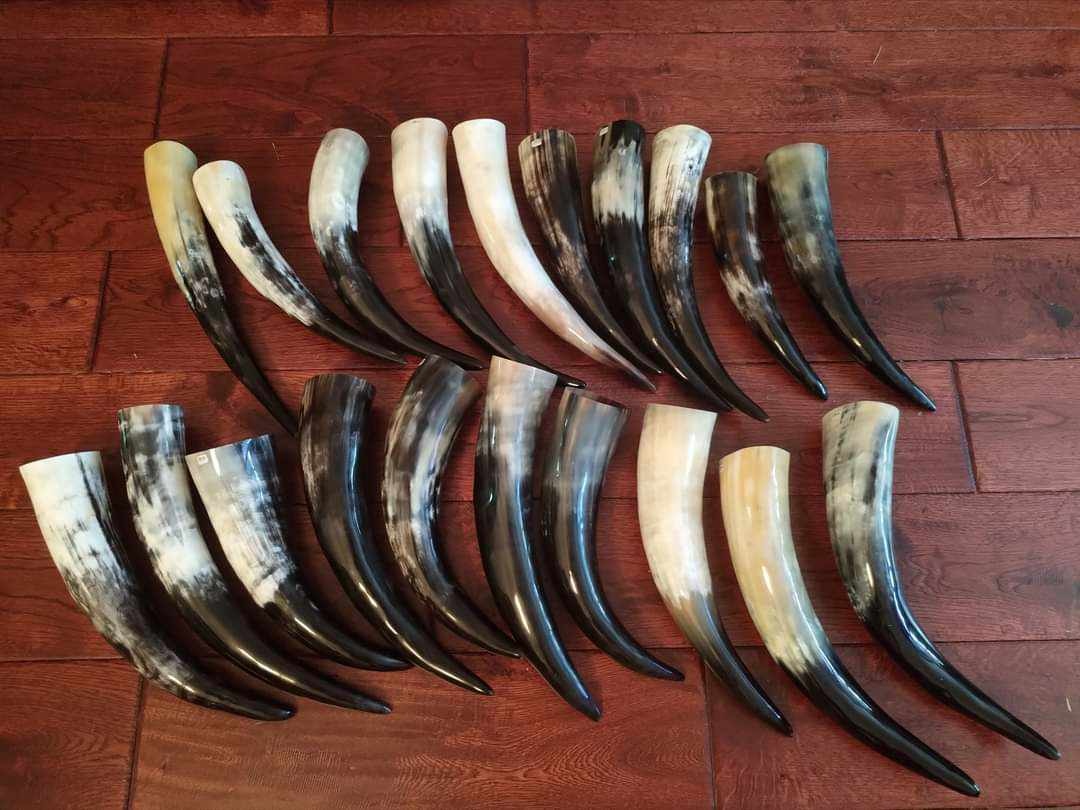The image showcases twenty highly polished animal horn-like structures arranged meticulously on a deep cherry-colored wooden floor. Organized into two parallel rows of ten, the horns vary in hue and size, with the top row featuring slightly smaller specimens compared to the larger ones on the bottom. The horns exhibit a striking array of colors, including variations of light tan, brown, dark brown, gray, white, and black. Most horns display a two-toned gradient, transitioning from a lighter base to a darker tip. Additionally, the cut edges of the horns are clean and straight, adding to their decorative allure. The overall scene emphasizes the diverse yet harmonious arrangement of these beautifully polished objects against the rich, warm tone of the wood.